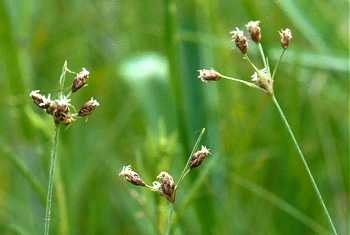A small image captures an outdoor scene bathed in subdued light, suggesting early morning or shaded atmosphere. In the background, tall, vibrant green grasses stand lush and dense. In the foreground, three stems rise, each adorned with buds transitioning from a delicate purple to a fresh light green, hinting at the imminent burst of new life. This intimate snapshot encapsulates the beauty of spring's arrival, inviting viewers to pause and appreciate the small wonders of the natural world.